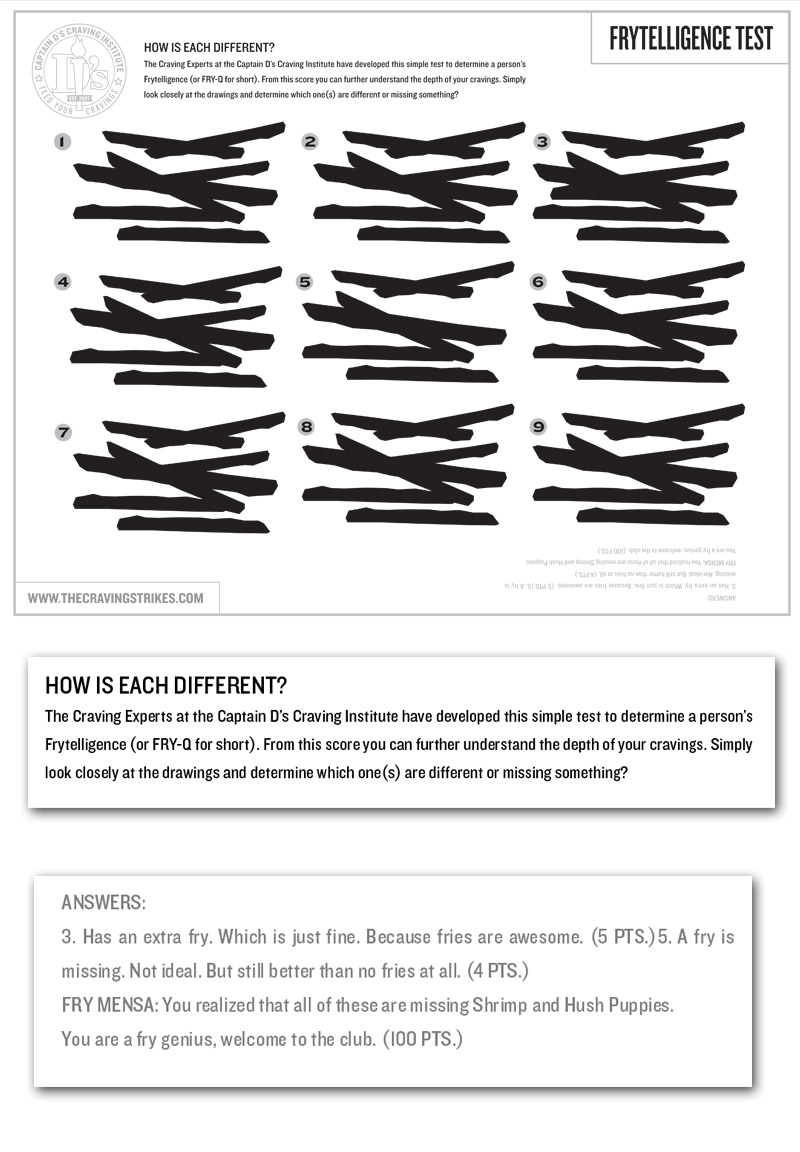The image is a compilation of three horizontally aligned rectangular sections, all featuring black drawings and text on a white background. The top section is titled "How is each different?" and labeled as a "fry intelligence test" on the upper right. It showcases nine black-and-white silhouette images of French fries, arranged in rows, each slightly different from the next. In this section, the Captain D's Craving Institute logo is displayed in the upper left, featuring a torch emblem and the text "D's" with "Established 2007."

The middle section reiterates the title "How is each different?" with a brief explanation stating, "The craving experts at the Captain D's Craving Institute have developed this simple test to determine a person’s fry intelligence, or fryQ for short. From this score, you can further understand the depth of your cravings. Simply look closely at the drawings and determine which ones are different or missing something."

The bottom section, highlighted in gray, is labeled "Answers" in the top left corner. It provides detailed feedback: for instance, "Number 3 has an extra fry, earning five points," and "Number 5, a fry is missing, earning four points." Additionally, a humorous note declares, "Fry Mensa, you realize that all of these are missing shrimp and hush puppies. You are a fry genius. Welcome to the club! A hundred points." At the very bottom, the image includes the URL: www.thecravinginstitute.com.